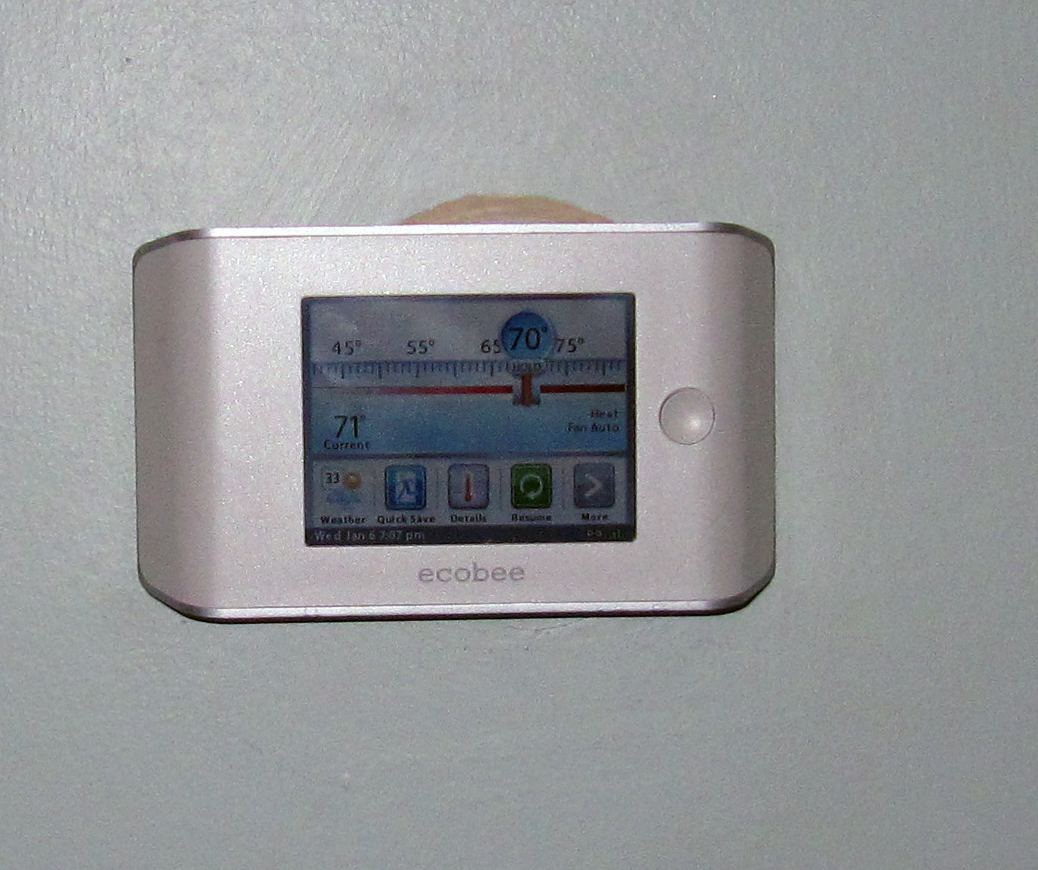A close-up of a wall painted in a sleek silver-gray hue reveals an electronic device prominently mounted on it. The device, resembling a modern thermostat, features a rectangular, silvery metallic body that blends seamlessly with the wall's elegant finish. At the center of the device, a small, clear screen displays a horizontal thermometer with a red line marking the current temperature. The thermometer scale ranges from 45 to 75 degrees Fahrenheit, with the current reading highlighted at 70 degrees. Below the thermometer display, there are various buttons that indicate options for weather updates and additional details, suggesting a multifunctional and user-friendly device.